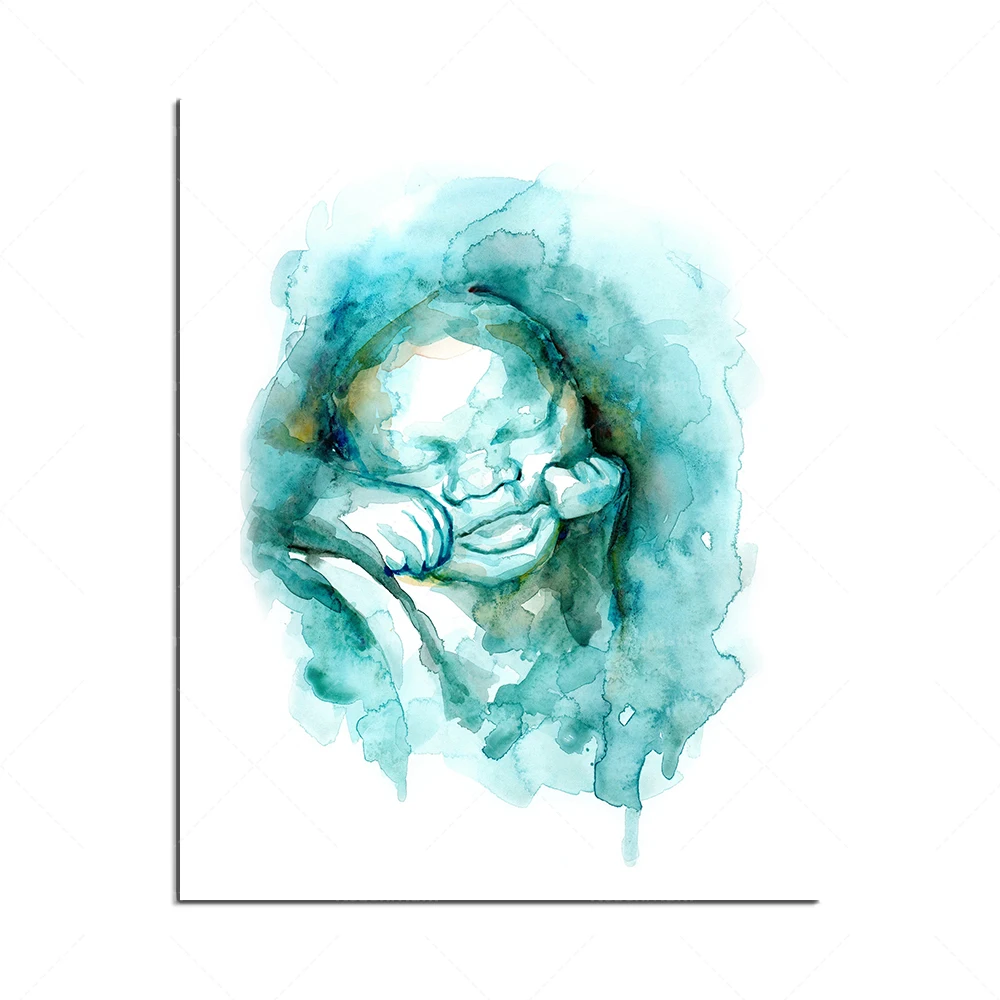This image showcases an artistic watercolor painting featuring a baby, set against a white background with a thin, black border along the bottom and left-hand sides. The painting is rectangular in portrait orientation and depicts a baby in hues of teal and light blue, with slight brownish-yellow accents near the forehead. The background appears white, blending seamlessly with the surrounding space, making it seem frameless.

Central to the artwork is the likeness of a baby, reminiscent of an ultrasound image. The baby’s eyes are closed, its mouth slightly open, and it has a broad nose. One hand, with its palm down and fingers curved, is positioned beneath the right cheek, near the mouth, while the other hand is tightly balled into a fist, pressed against the baby’s left cheek. The proportions and positioning suggest a sense of comfort and tranquility, as if the baby is peacefully dreaming.

The overall color palette features varying shades of blue, giving the piece a fluid, runny appearance characteristic of watercolor paintings. The teal hues dominate the baby’s head and flow downwards, bleeding into the white canvas in a lighter shade at the top, creating a gentle contrast. The blue splotches surrounding the baby add an abstract, swaddled effect, enhancing the ethereal quality of the artwork.